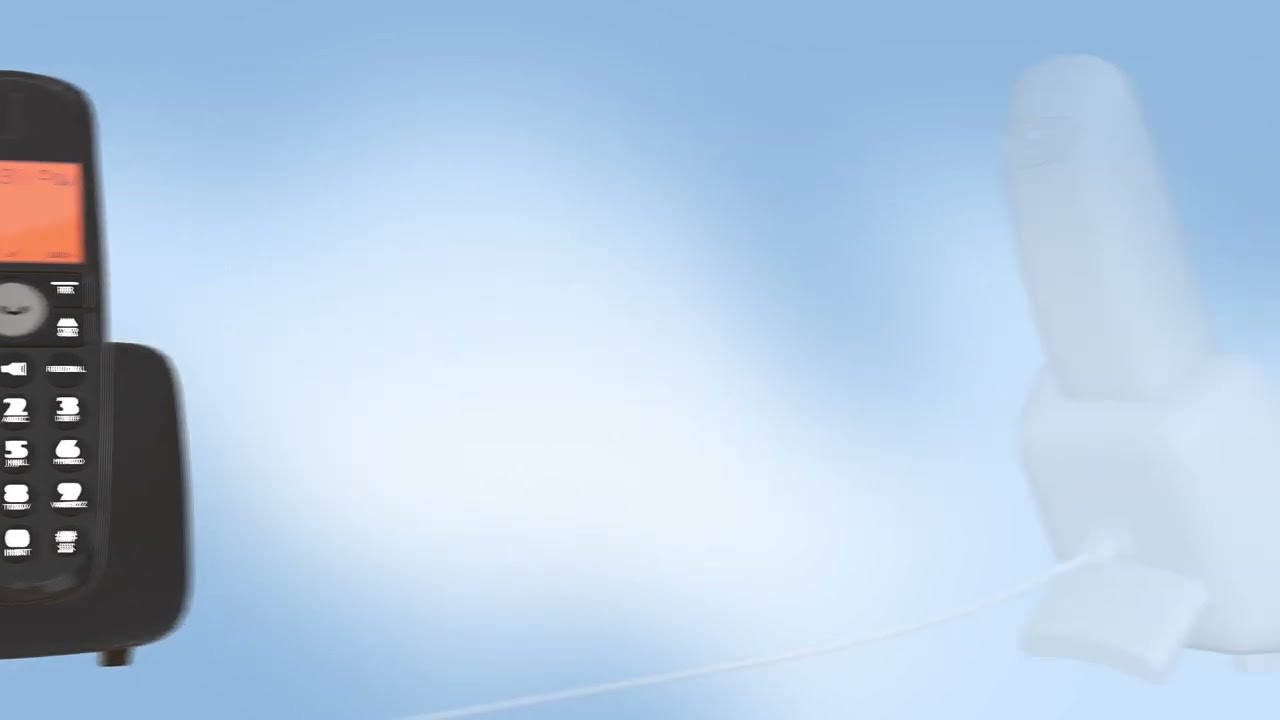The image features a horizontal graphic with a cloud-like gradient background, transitioning from white in the center to sky blue at the edges. Central to the composition are white bulbous regions that blur into the gradient backdrop. On the left side of the graphic, there is an old-fashioned black corded phone resting in its cradle, with a prominent orange digital display screen and white keypad lettering. Below the screen is a round gray button featuring a phone icon in profile. This handset evokes the style of phones from the 80s or 90s and sits on a black docking station. On the right side of the graphic is a white plastic object, semi-transparent and blurry. It appears to be a base unit matching the black handset, with a large switch at the bottom and an additional object resembling a small building atop it. A white power cord extends from the back of this right-sided object towards the left, connecting to the cradle of the black phone.